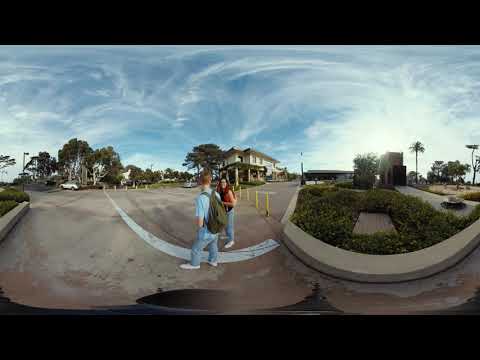In this detailed panoramic color photograph, there is a horizontal black stripe across the top and bottom, framing a composite image created with special fisheye and panorama filters. The scene captures a parking lot where two people, a young man, and a young woman, are walking and conversing. The young man on the left sports a light blue short-sleeved shirt, a green backpack, blue jeans, and white sneakers, with his hands casually tucked into his pockets. To his right, the young woman wears a red shirt, blue jeans, and white shoes.

The background features a mix of natural and urban elements under a bright blue sky adorned with wispy, feathery white clouds. To the left, there's a curb beside a landscaped area of green bushes and grass, along with a gray sidewalk. Several yellow traffic pylons are visible behind the couple, serving as barriers. Further back, trees with brown stems and branches frame a white house with brown roofing, adding a residential touch to the scene.

To the right, beyond a concrete curb, a landscaped yard leads to another building flanked by palm trees. The overall composition blends urban and suburban elements, suggesting the setting could be a school, residential area, or tourist location, blending everyday life with a touch of artistic photographic techniques.